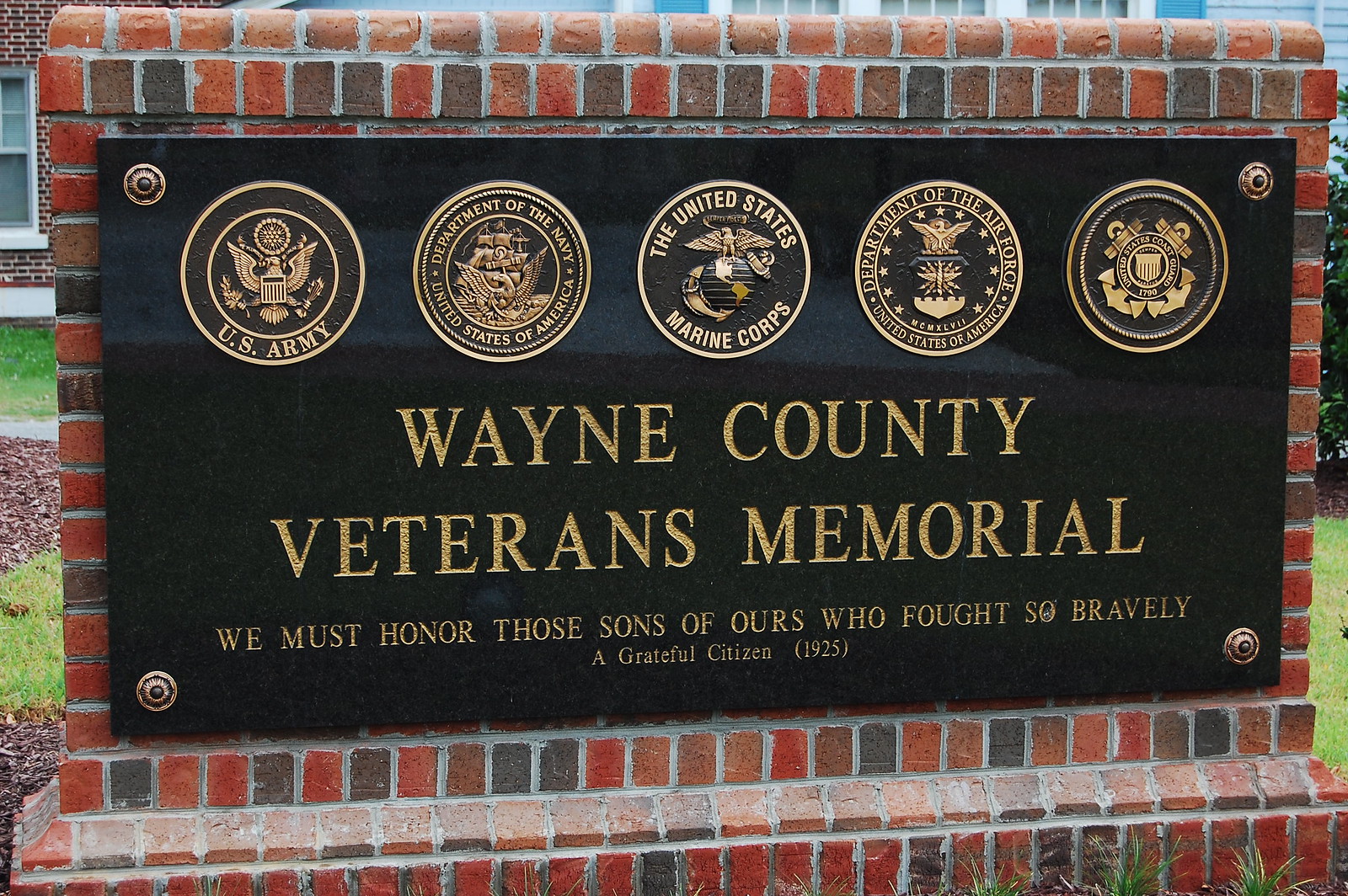In this wide rectangular image, a prominent black marble sign is affixed to an expansive brick wall comprised of small, alternating square-shaped bricks in reddish, dark grayish-brown, and orangey-brown hues. This sign, which serves as the Wayne County Veterans Memorial, is bordered by lush green grass lawns and mulch piles on either side, while above, portions of a brick building with white windows are visible. The sign features five circular, gold insignias at the top, each representing different branches of the military: the U.S. Army, the Department of the Navy, the United States Marine Corps, the Department of the Air Force, and the U.S. Coast Guard. Below these insignias, gold, all-capital letters spell out "WAYNE COUNTY VETERANS MEMORIAL." Directly beneath that, in a smaller font, the inscription reads, "We must honor those sons of ours who fought so bravely, a grateful citizen, 1925." The sign is secured into the brick wall with noticeable gold bolts at each corner, adding to its dignified and solemn appearance.